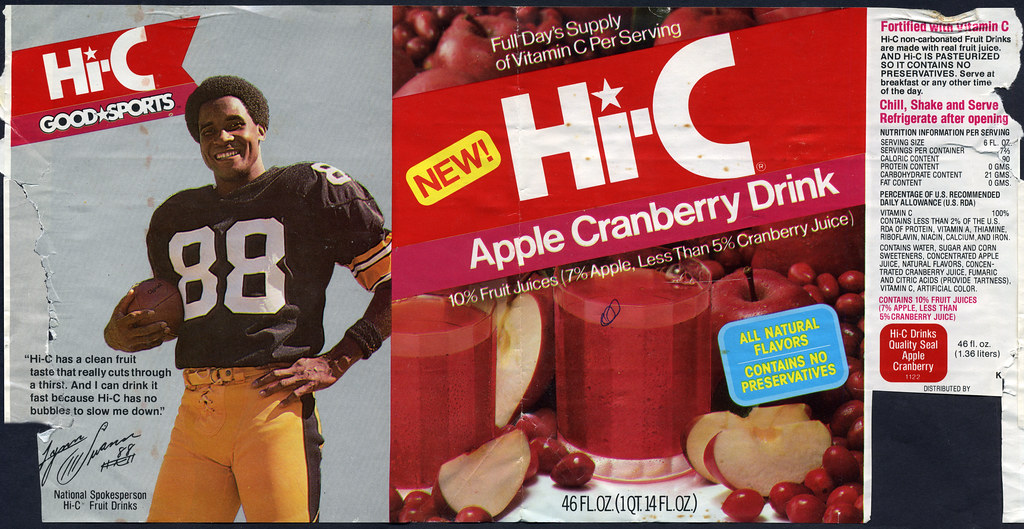The image features a vibrant Hi-C label, prominently displayed with large white letters on a bold red background. A yellow bar at the top of the label announces "New," and a pink bar at the bottom states "Apple Cranberry Drink" in white letters. A glass filled with the drink is pictured, surrounded by illustrations of apples and cranberries, enhancing the fruity theme.

To the left, a gray section displays the Hi-C logo again, in striking red and white. Adjacent to this, a smiling football player dressed in a black and yellow uniform poses confidently, holding a football at his side.

On the right side of the image, a white panel features small pink and black text, providing additional information in a concise format. At the bottom of this section, viewers are directed to visit www.FEMA.gov for more information.